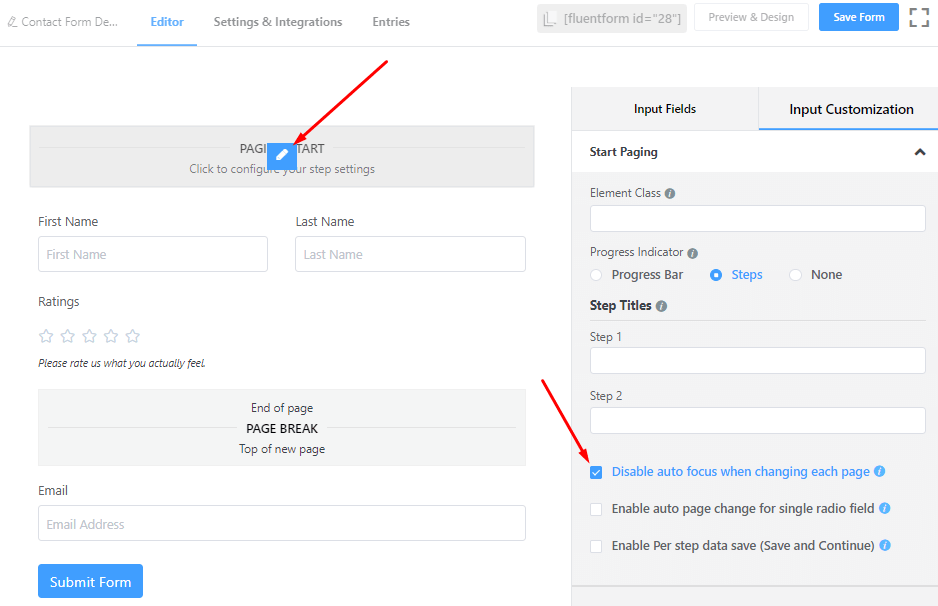This is a screenshot from an unknown source showcasing a form editor interface. At the top, there is a menu bar with multiple options: "Contact Form," "Editor" (which is selected), "Settings and Integrations," "Entries," "Fluent Form ID," "=", "\"28\""," "Preview and Design," and "Save Form." On the left side, a gray banner displays the text "Paging Start, click to configure your step settings" with a blue square icon partially obscuring the text. The blue square features a white pencil icon, signifying edit functionality. A red arrow has been added, pointing to this blue icon, indicating its significance.

Below this, the form fields begin with "First Name," "Last Name," and "Ratings," indicated by four white stars accompanied by the text "Please rate us what you actually feel." Following a "Page Break," the next page includes fields for "Email" with placeholders for "Email Address" and a "Submit Form" button.

On the right side of the interface, there are options for "Input Fields" and "Input Customization," with "Input Customization" currently selected. The customization panel lists options like "Start Paging," "Element Class," "Progress Indicator," and "Progress Bar." The "Steps" section is highlighted, displaying "None," "Step Titles," "Step One," and "Step Two." A checkbox with the label "Disable auto focus when changing each page" is checked, indicated by a red arrow pointing to it. Additional settings include "Enable auto page change for single radio field," "Enable per step data save," and "Save and Continue."